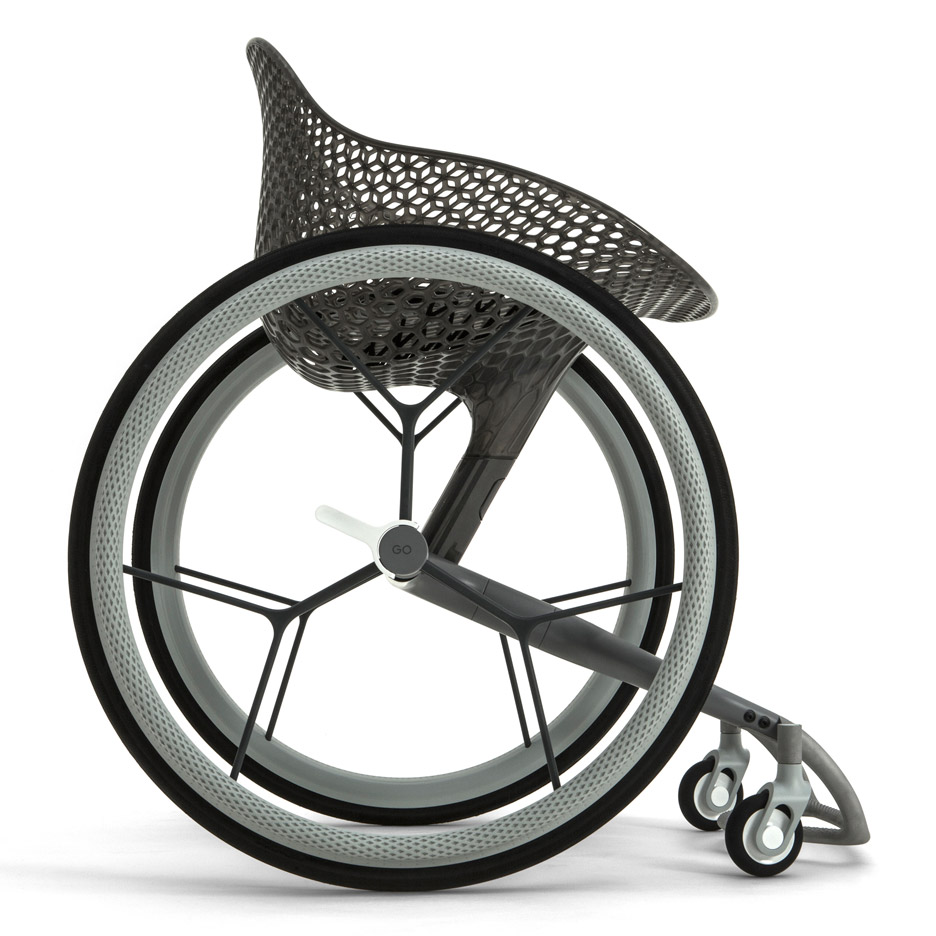This is a detailed illustration of a unique wheeled apparatus, likely designed for individuals with mobility challenges. It features two large black wheels, resembling oversized bicycle or wheelchair tires with gray white-wall accents, positioned side by side. The wheels are connected by a metal or fiberglass post, forming the central axis of the device. In the front section, two smaller black wheels are attached, which appear to aid in stability and steering. These smaller wheels are connected to a gray bar and a fork-like structure.

The device includes a gray bucket seat with a mesh or honeycomb pattern, providing a breathable and supportive seating area. Notably, the seat lacks restraints such as seat belts or straps. The overall design suggests that users propel themselves forward while seated. The frame consists of thin, grayish metal bars arranged in a triangular pattern, contributing to the sturdy yet lightweight construction of the apparatus. The entire setup is depicted in a black-and-white drawing with no explanatory text, leaving its specific purpose open to interpretation.